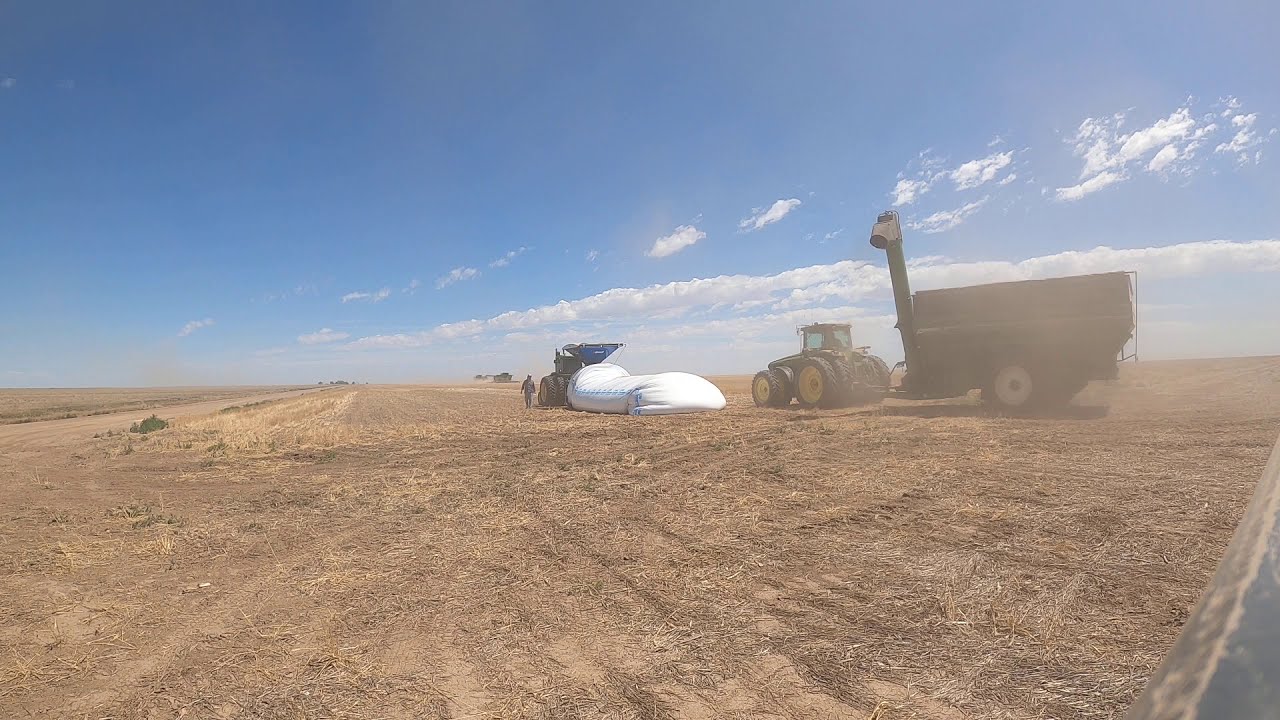In this image, we observe a vast and flat expanse of farmland, primarily comprised of bare, dirt-covered ground, indicative of a recently harvested field, possibly a cornfield. Dominating the scene are two tractors engaged in farming activities. The tractor on the right is pulling a large white object that resembles a giant sack or storage container. On the left, another tractor with a man standing beside it is visible. In the middle background, there's a haze, presumably from the active machinery. The sky above is a brilliant blue adorned with a series of white clouds - some form a stream stretching across the horizon, while others are sporadically scattered. There's a hint of a dirt road on the left side in the background, and the top half of the picture vividly captures the bright daylight. The overall atmosphere is one of intense agricultural activity under a clear and spacious sky.